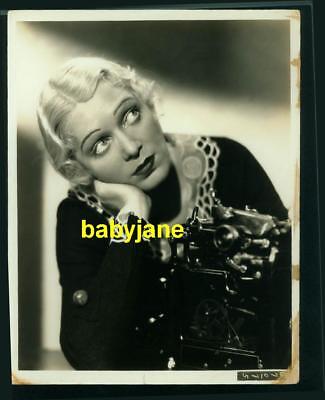This is a framed black and white photograph of a woman from the 1920s, likely an actress. The white frame is surrounded by a black border, and the image itself shows some signs of water damage. The woman has short, platinum blonde, wavy hair parted to the side, and she wears a black dress with a white mesh-like collar. Her makeup includes very thin eyebrows, mascara, and lipstick, which accentuate her features. She is leaning forward, resting her cheek against her right palm, and gazing upward and to her right. A camera or recording device is visible in the bottom right corner of the image, along with an unclear object on what appears to be a table in front of her. There is yellow text in the center of the photo that reads "baby jane" in lowercase letters.